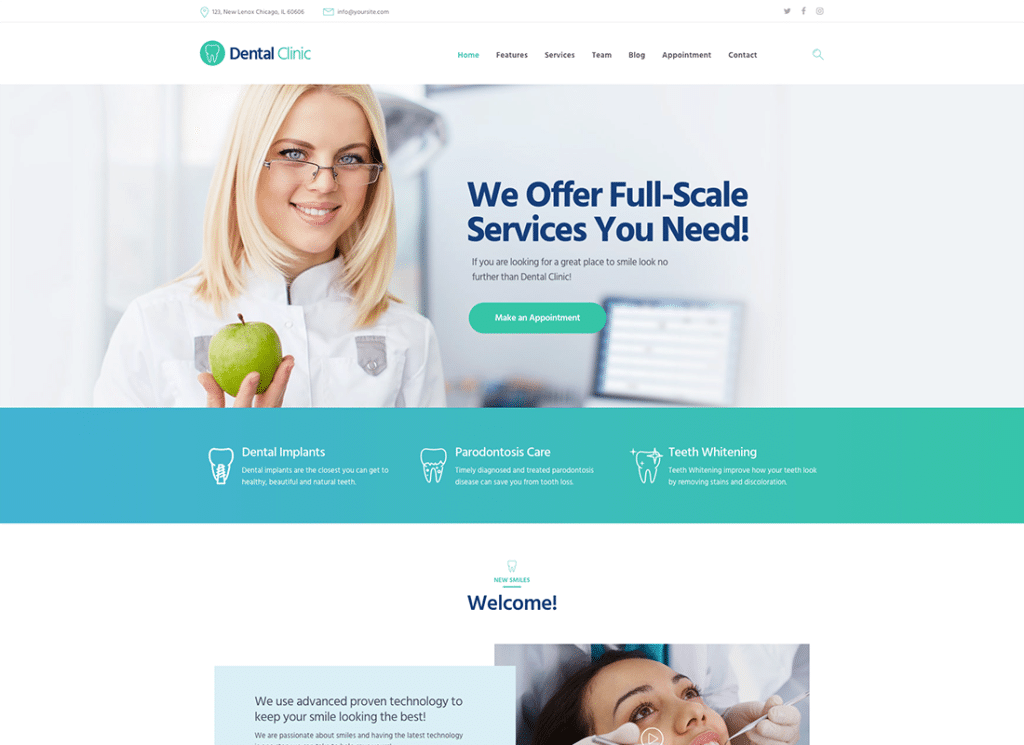The image depicts a webpage layout for a dental clinic, aimed at presenting the clinic's offerings and inviting user interaction. 

In the upper left corner, the screen displays the text "Dental Clinic". The header menu includes the following navigation options: "Home," "Feature," "Services," "Team," "Blog," "Appointment," and "Contact," with a magnifying glass symbolizing the search function. 

Below the header, there is a prominently placed photograph of a woman with blonde hair and glasses, holding a green apple. She has blue eyes and is wearing a white shirt, looking directly at the camera. 

To the right of her image, blue text states, "We offer full-scale services you need." Beneath this, a small paragraph in black text provides additional details. Further down, there's a green button with rounded edges and white text reading, "Make an Appointment."

Descending the page, a section features a gradient background transitioning from blue to teal green, which serves as a visual separator. Below this gradient section, another area declares "New Smiles Welcome" over a light blue background with black text.

On the right-hand side of this section, there is an embedded video showing a woman receiving dental services.